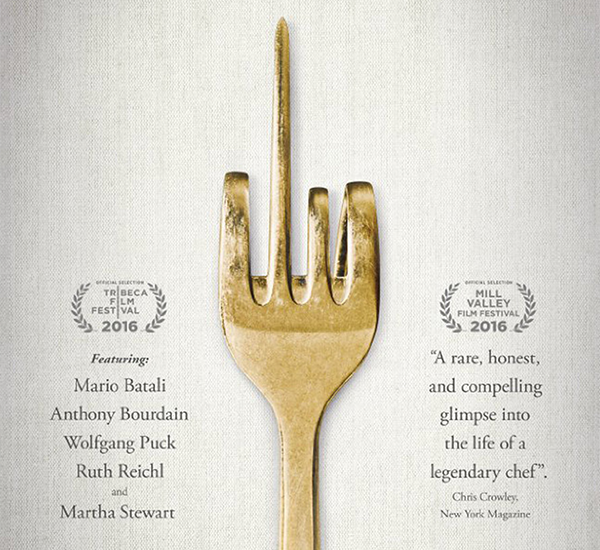The film poster features a textured gray background, presenting a gradient that transitions from lighter gray at the center to darker gray towards the edges. Centrally positioned, a gold fork stands out with its unique design—three prongs bent down while the second prong from the left remains upright. Gray, semi-transparent text accompanies the fork on both sides. On the left, the text reads "Tribeca Film Festival 2016, featuring Mario Batali, Anthony Bourdain, Wolfgang Puck, Ruth Reichl, and Martha Stewart." On the right, the text announces, "Mill Valley Film Festival 2016, a rare, honest, and compelling glimpse into the life of a legendary chef," attributed to Chris Crowley of New York Magazine. The fork extends towards the bottom edge, perfectly centered alongside the equally centered textual elements, evoking an intriguing and minimalist aesthetic to advertise an upcoming film festival.